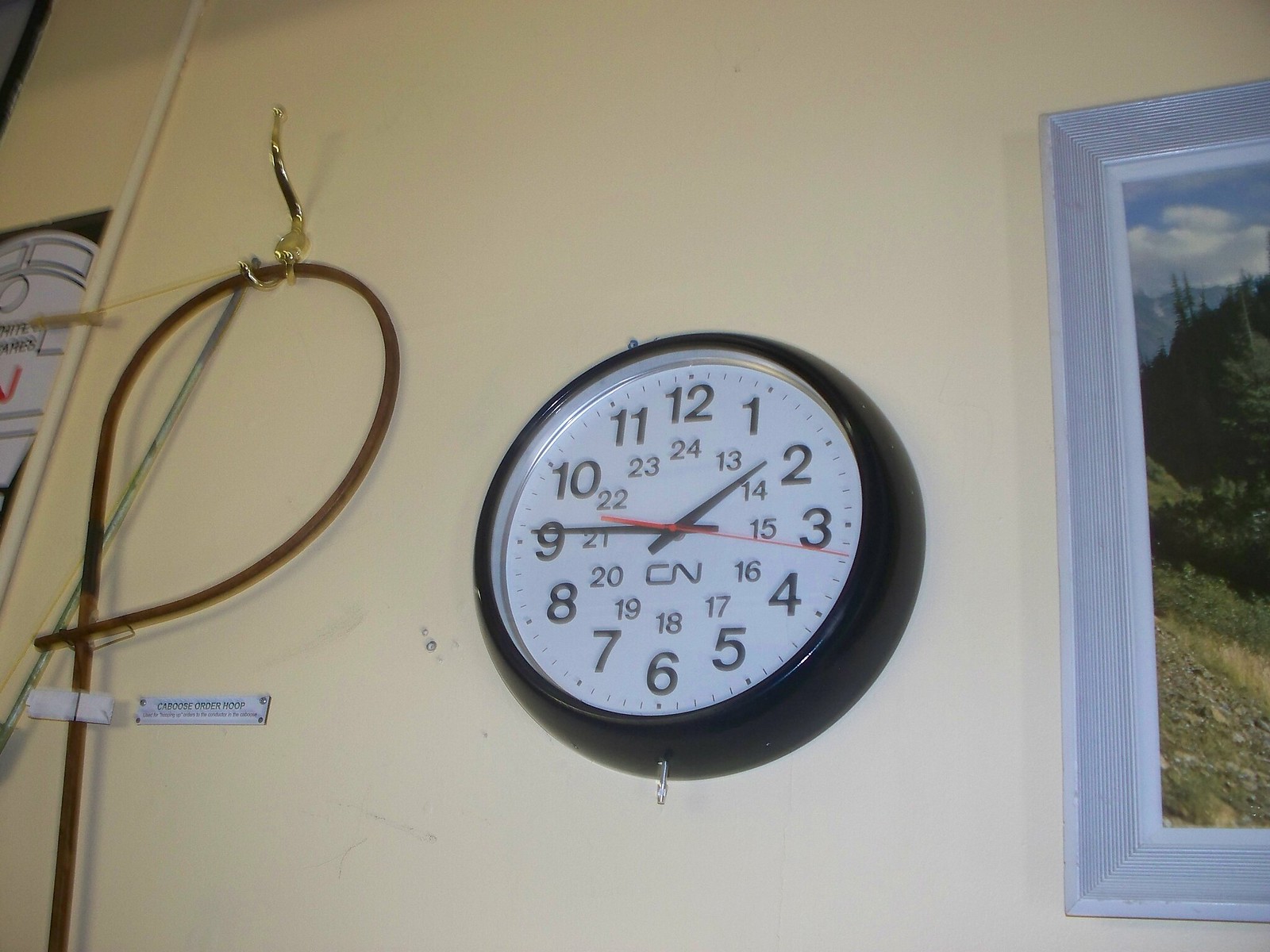In the image, a cream or pastel yellow colored wall serves as the backdrop. On the left-hand side, a gold-tone coat hanger is bolted to the wall, with a brown cord looped around it. Just to the right of the cord hangs a small white tag with black writing, tacked to the wall with silver-tone tacks or screws. The tag reads "Caboose Order Hoop." 

In the center of the wall, there is a round black and white clock. The clock features a white face with black numbers marking 1 through 12 and smaller black numbers marking 13 through 24 for military time. The clock’s hands include a short black hour hand, a long black minute hand, and a thin red second hand. Underneath the hands, the letters "CN" are printed in black, and the clock is encased in a black frame.

To the right of the clock is a light blue painted picture frame with a ridged texture, containing a painting or photograph of an outdoor scene with green trees, bushes, grass, and a blue and white cloudy sky. This image completes the composition on the pastel-colored wall, combining both functional and decorative elements.